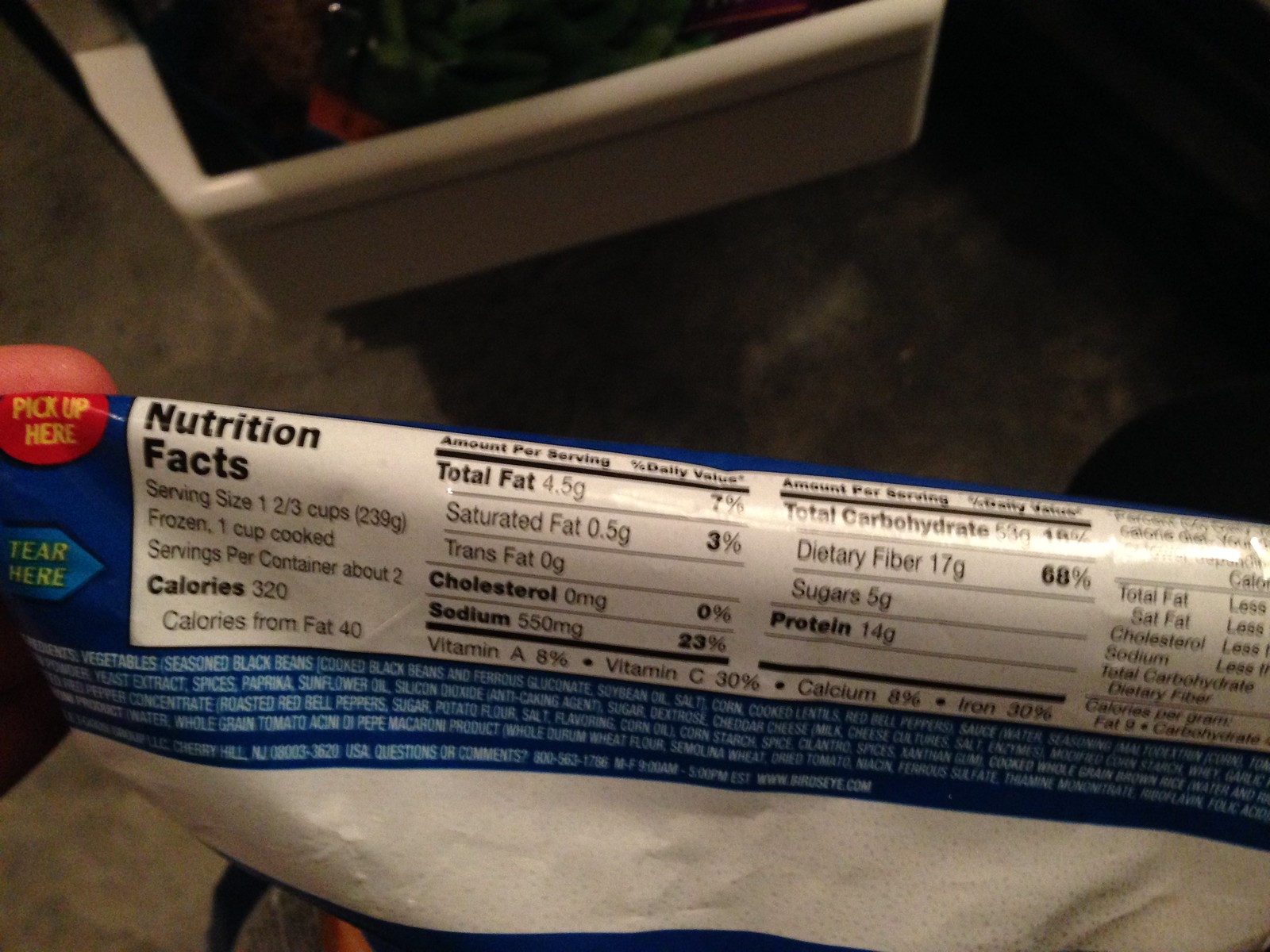Nutritional information on a plastic package is visible. The package is predominantly blue with white labels. In the background, there is a table at a distance and another container, which contains something cream-colored in its center. On the left side of the package, there is a red circle at the top that says "Pick up here" and a blue arrow pointing to the right that instructs "Tear here." This package contains vegetables, seasoned black beans, soybean oil, and corn. The serving size is one and two-thirds cups when frozen and one cup when cooked, delivering 320 calories per serving. There are approximately two servings per container.